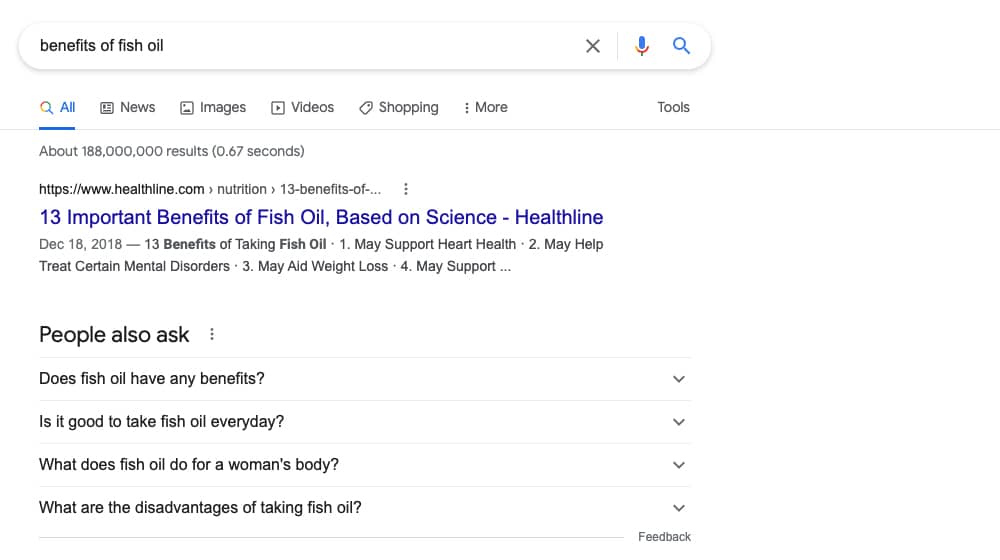In this detailed image, we observe a Google web search page. Dominating the upper section is the familiar elongated search bar, prominently displaying the query, "benefits of fish oil." Adjacent to the right end of the search bar, a small gray 'X' button allows for quick deletion of the typed text. To the right of the 'X' is a multicolored microphone icon in Google’s signature blue, red, yellow, and green hues, indicating the option for voice search. At the far right, a blue magnifying glass icon invites the user to initiate their search.

Below the search bar, various navigational tabs are arranged horizontally: 'All,' which is highlighted in blue, followed by 'News,' 'Images,' 'Videos,' 'Shopping,' and a 'More' dropdown option. Alongside these tabs is a 'Tools' button situated towards the right-hand side of the screen.

Directly beneath the navigation tabs, the search results indicate that approximately 188 million results have been found, impressively compiled in just 0.67 seconds. The first search result is a blue hyperlinked title, "13 Important Benefits of Fish Oil Based on Science," attributed to the reputable source, Healthline. The associated web address is www.healthline.com. 

The image also includes a section titled "People Also Ask," featuring frequently asked questions such as, "Does fish oil have any benefits?" and "Is it good to take fish oil every day?" This layout provides viewers with a comprehensive glimpse into the depth and breadth of information available on the topic of fish oil benefits, alongside options for further exploration through additional queries and navigational tabs.